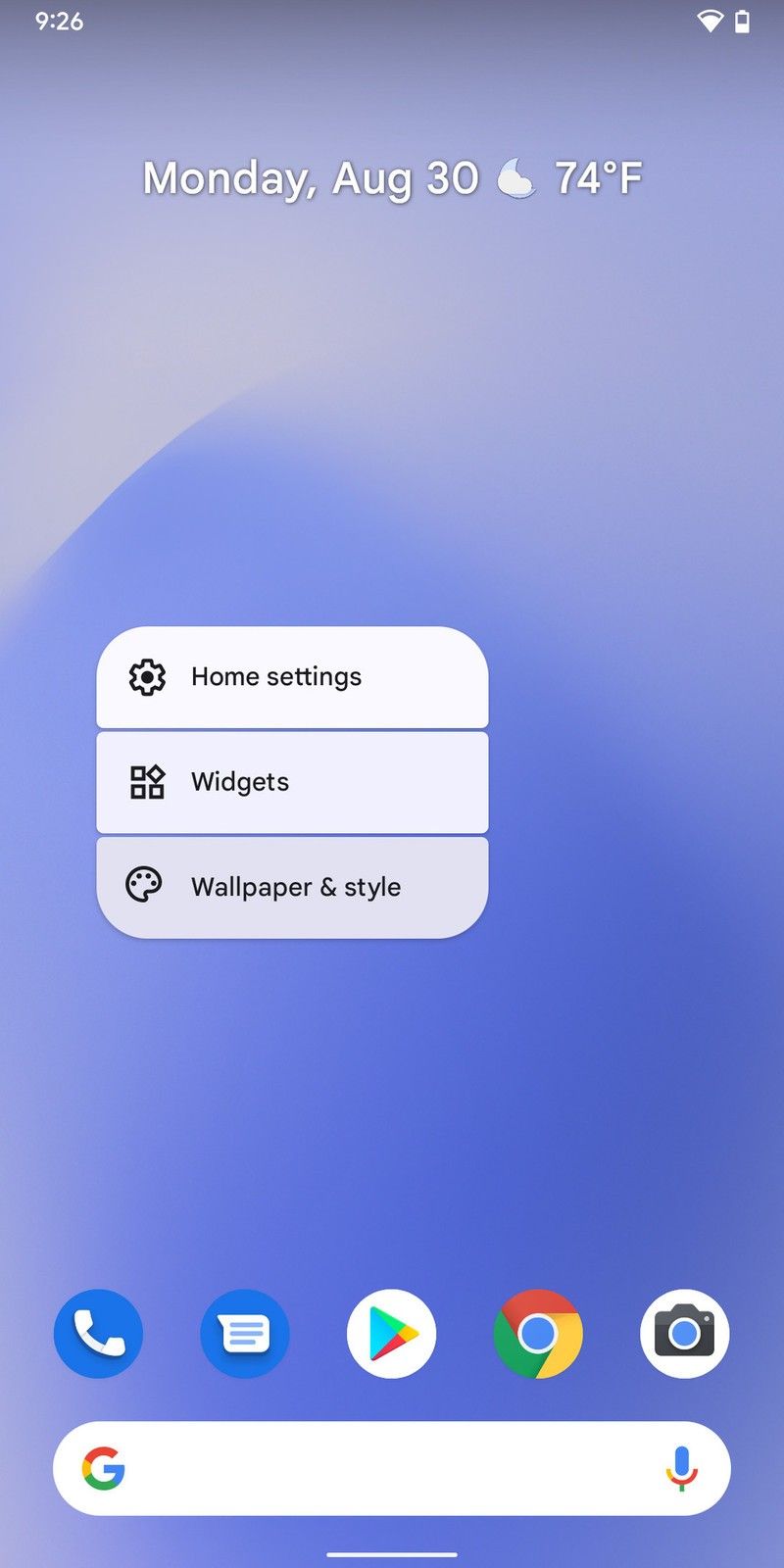A detailed screenshot from a smartphone's home screen, featuring a gradient background that transitions from a purple, fog-like appearance at the top to a blue, mountainous impression at the bottom. In the upper left corner, the time is displayed in white text as "9:26," while the upper right corner features white icons for battery and Wi-Fi status, with the battery showing approximately 50% charge. Centered just below these icons, the date "Monday, August 30th," the temperature "74°F," and a small white cloud icon are arranged, creating a clean, informative header.

Beneath this header, a rectangle with rounded corners and a light lavender hue houses options such as "Home settings," "Widgets," and "Wallpaper and style," each separated by a thin gray line. At the bottom of the screen, a white, rectangular search box with rounded corners features the Google logo on the left and a microphone icon on the right, indicating voice search capability. Above this search box, icons for essential apps like Phone, Messages, Google Play Store, Google Chrome, and Camera are neatly organized, completing the coherent and functional layout of the smartphone's home screen.